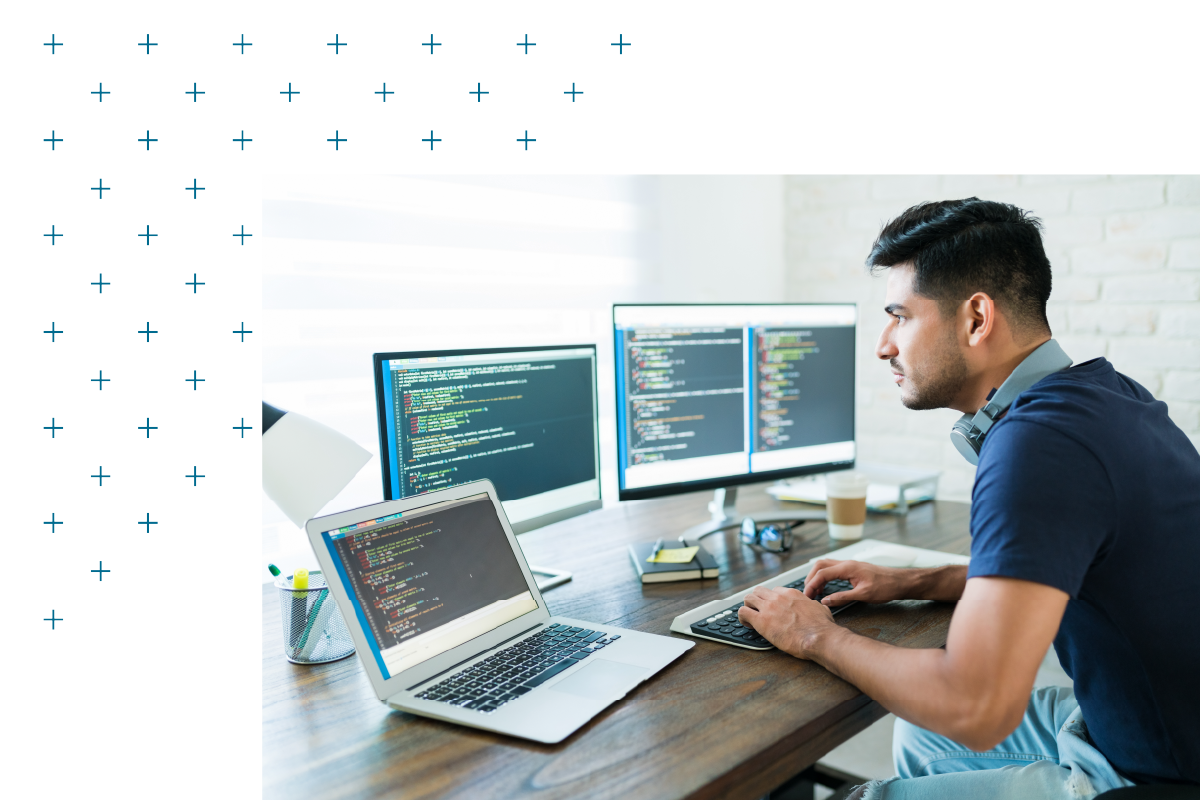The image features a white background with a graphic series of dark and light blue plus signs forming a triangular pattern in the upper left corner. On the lower right side, a man with black hair and gray headphones around his neck is seated at a darker wood grain desk, typing on a black keyboard with a gray base. He is dressed in a dark blue shirt and blue jeans. The desk holds an open silver laptop displaying code in red, white, and yellow on a black screen. Behind the laptop are two computer monitors, both displaying code in various colors; one monitor has a black frame with a silver bottom, while the other has a black frame with white top and bottom sections. Positioned in front of the monitors are a pair of reading glasses, a small black notebook with a yellow sticky note, and a white coffee cup with a brown cardboard sleeve. On the left side of the desk, there's a desk lamp and a mesh metal container holding pens and markers. The setting resembles a modern, focused workspace, capturing the essence of someone engrossed in their coding tasks.